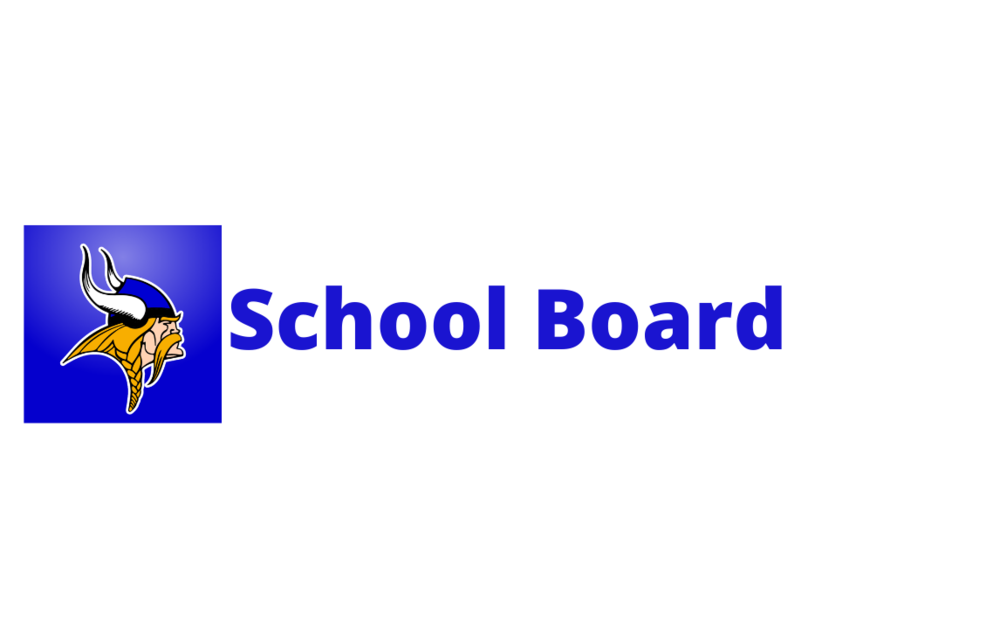The image features a prominent logo and text set against a wide expanse of empty white space. On the left, there is a square logo with a blue background, depicting a Viking head. The Viking, characterized by his long, possibly braided brown hair, has a pointed chin, bushy brown eyebrows, and a long brown mustache. He looks serious and is gazing off to the side. The Viking wears a purple hat with a black border, and two white horns that have black tips. To the right of the logo are the words "School Board," written in large blue letters with each word capitalized at the beginning. The overall composition features a lot of blank white space above and below the central elements, focusing attention on the logo and the text.